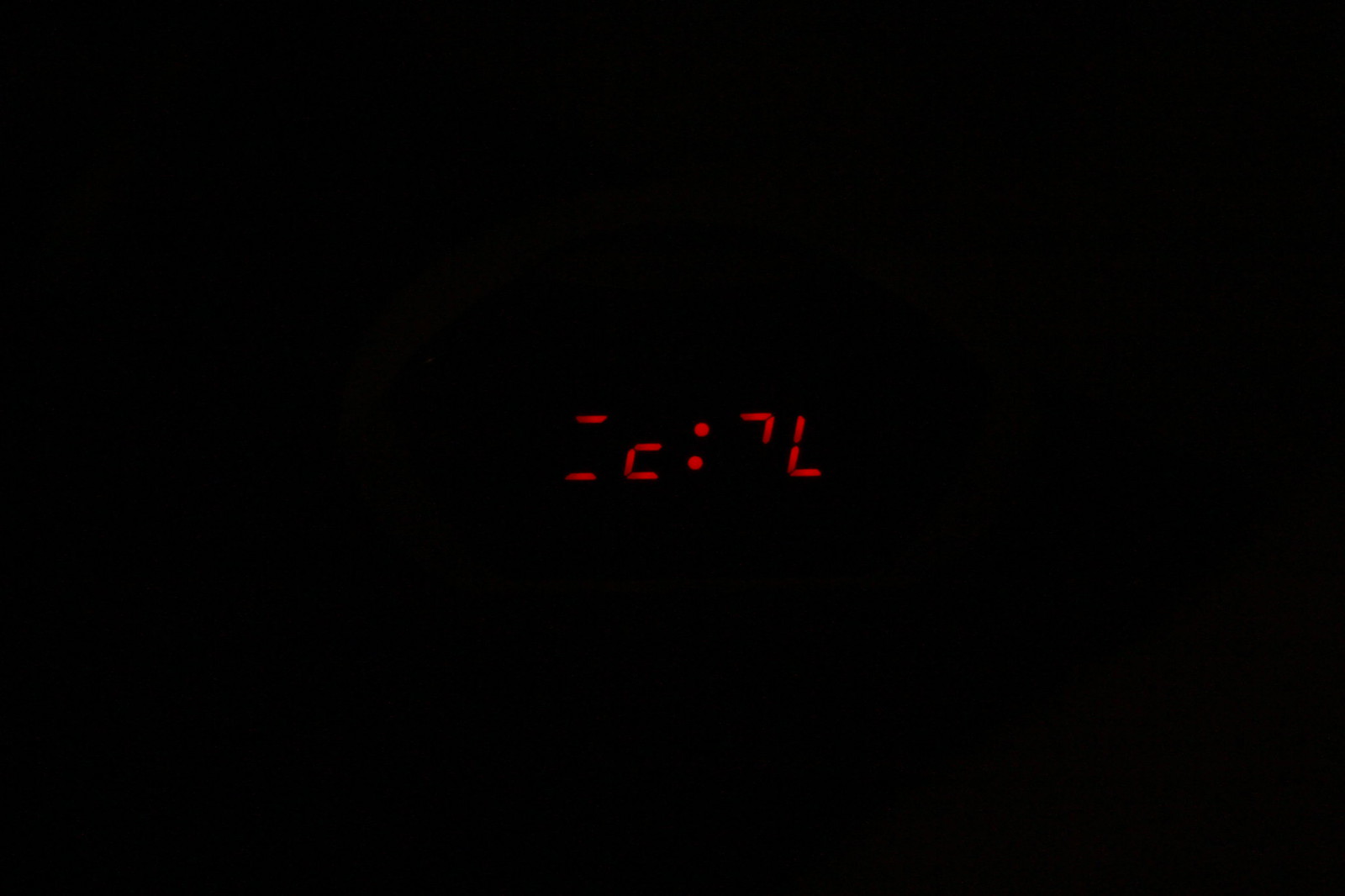In the center of this image, set against a stark black background, are a series of small, bright red characters. The characters are arranged horizontally, starting on the left with two dashed lines. Following this, there is a lowercase "c," succeeded by two vertically stacked dots. Next in the sequence is a tiny number "7," and finally, an uppercase "L." This arrangement of symbols is isolated, occupying roughly 5% of the entire image, with the inky blackness of the background encompassing the remaining space from edge to edge.